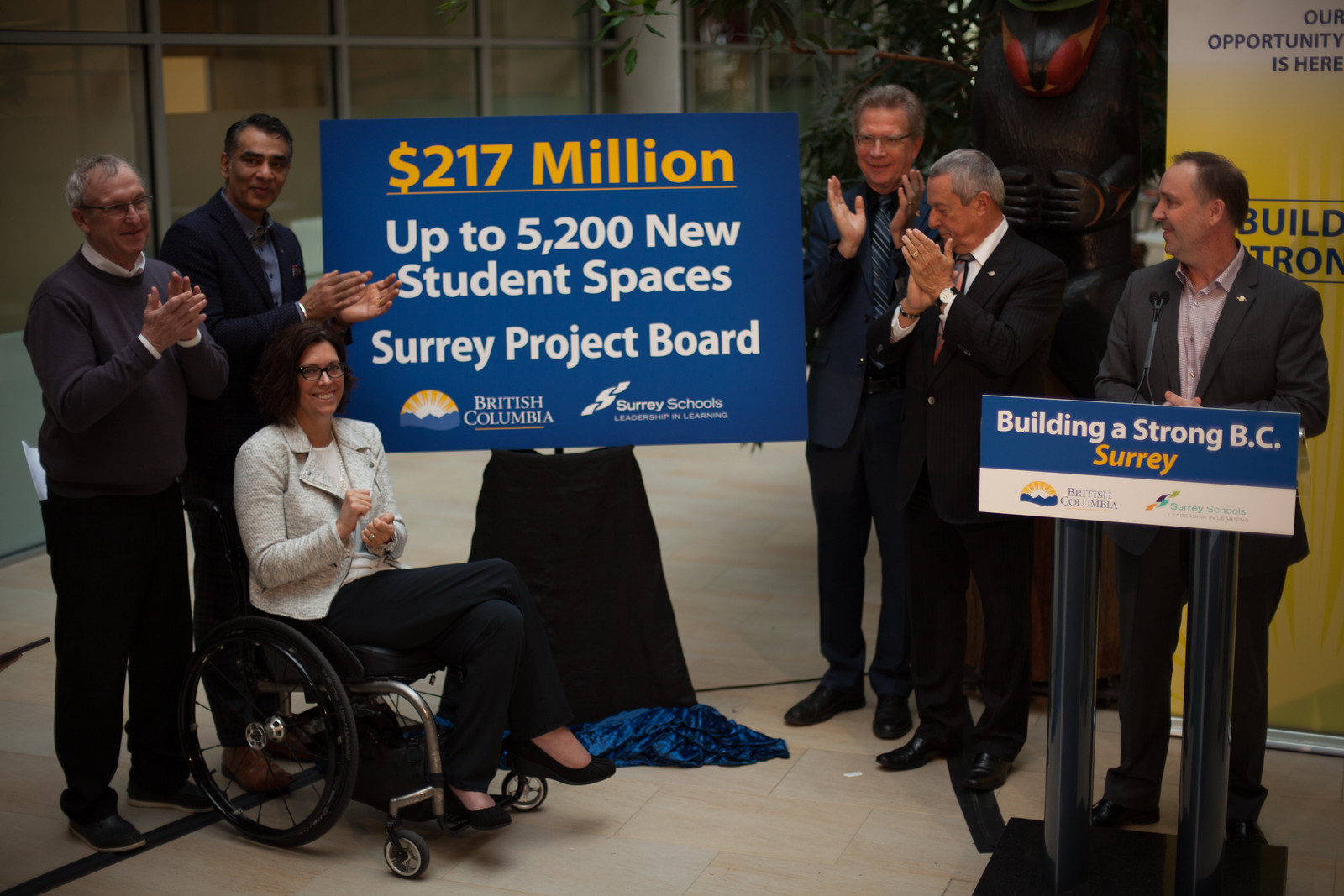The image depicts an indoor event, likely a conference or awards ceremony, featuring multiple individuals involved in an announcement. At the bottom of the screen, a tile floor is visible. Central to the image, a large sign with a blue background and the text "$217 million up to 5,200 new student spaces, Surrey Project Board, British Columbia, Surrey Schools" prominently displayed. This sign is key to the event and is highlighted in yellow, white, and orange print.

To the left of the sign, three individuals are visible: a woman in a wheelchair with short brown hair, dressed in black slacks and a white jacket, clapping, and two men in long-sleeved shirts, one of whom is also in a suit jacket. They have slightly tanned skin and are positioned behind the woman, also clapping and looking towards the right side of the image.

In the center-right of the image stands a man at a podium, with a sign on the front that reads "Building a Strong BC Surrey" in white and orange print. He is not clapping but is facing and looking slightly towards the left side of the image. To his left, two more men in business suits are also seen clapping.

The color scheme of the scene includes tan, blue, white, yellow, gray, black, and red. The overall composition illustrates a formal gathering rooted in significant community and educational development within British Columbia, emphasizing the financial commitment and expansion efforts in Surrey Schools.